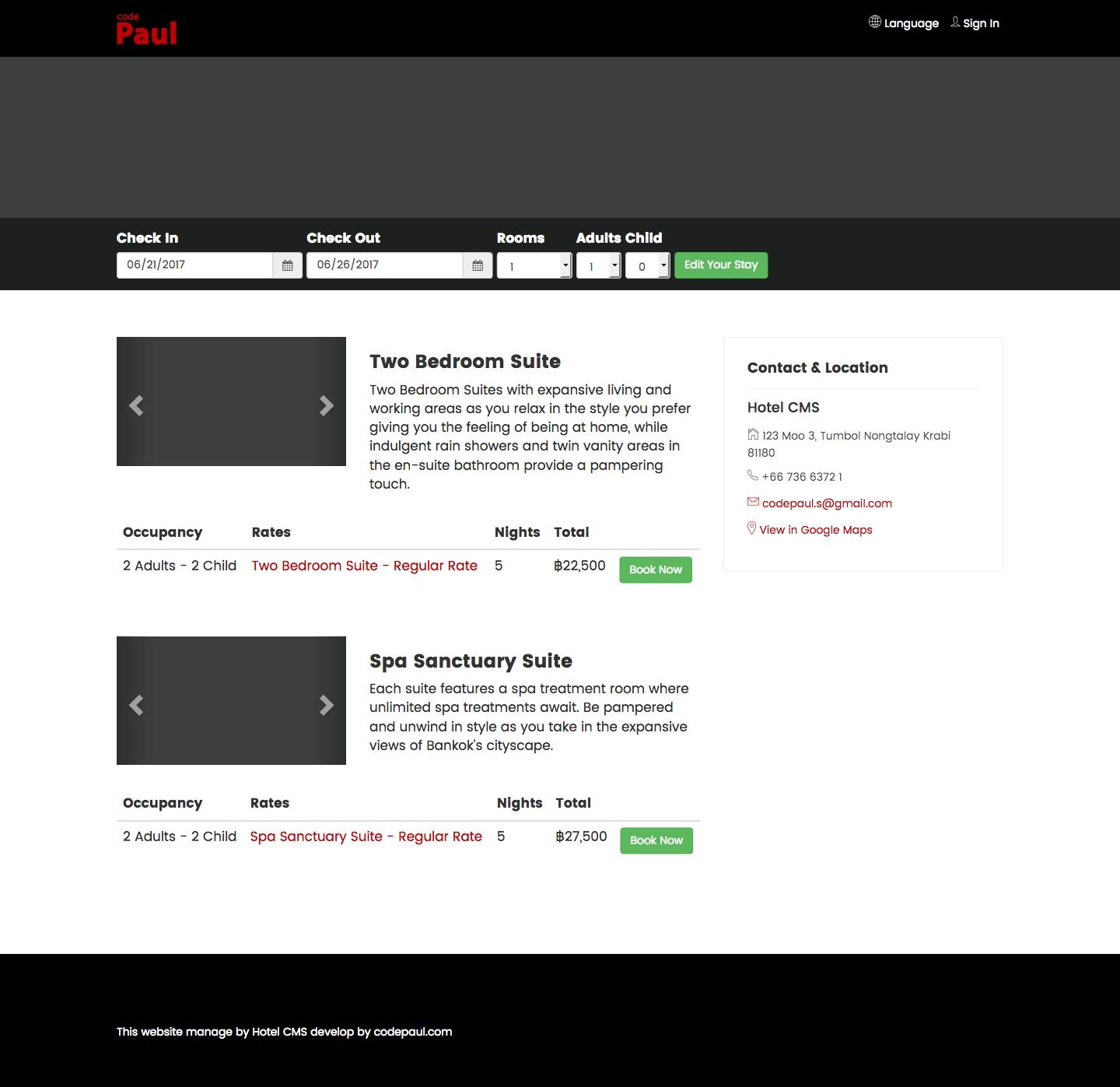The background of the top image is decorated with black stripes, and a black stripe runs prominently across the top. In bold red text, the name "Paul" is displayed. To the right, in very small text, are the words "Language" and "Sign In." 

In the center of the image, there is a large gray area containing the check-in details. It lists the check-in date as 06-21-2017, and the check-out date as 06-26-2017. It mentions that there is one room reserved for one adult and zero children. A green option is available to edit your stay.

Below that, two room options are presented. The first is a Two-Bedroom Suite, which features expansive living and working areas for a homely feel, while the indulgent rain showers and twin vanity areas in the en-suite bathroom add a pampering touch. This suite accommodates two adults and two children and costs B22,500. There is an option to "Book Now."

The second option is a Spa Sanctuary Suite, which includes a spa treatment room where unlimited spa treatments are available. Guests can unwind in style while enjoying expansive views of Bangkok's cityscape. This suite is priced at B27,500, with a "Book Now" option available.